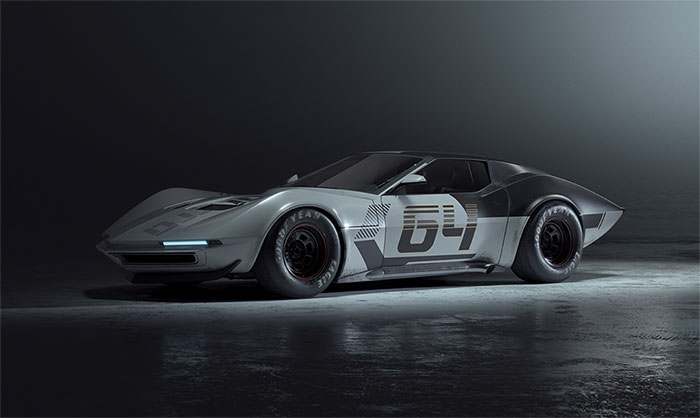This is a professional, black-and-white photograph of a sleek, luxurious sports car, reminiscent of the Batmobile, showcasing both sharp and smooth angles. The car, predominantly gray with black accents on the top, windshield, and one wheel, is marked with the number "64" on the door and features various decals. The tires, emblazoned with white "Goodyear" lettering, are prominently displayed. The setting includes a dark, gray-scale background that enhances the car's presence under a spotlight. Bright lighting in the top right of the image and around the car contrasts with the otherwise dark scene, drawing attention to the car's meticulous design and elegant form.